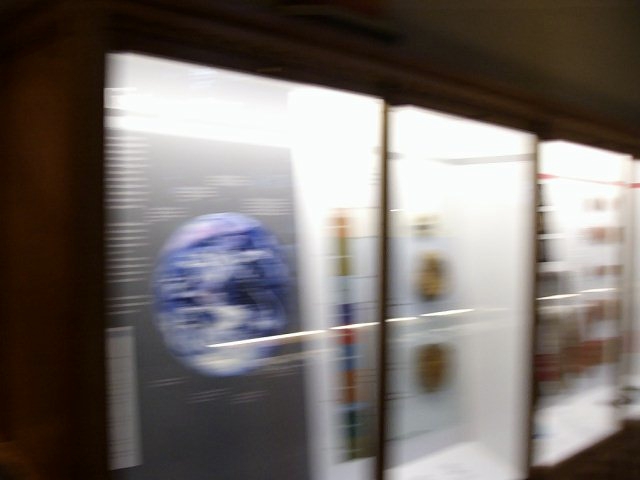The photograph is a very blurry image of what appears to be a museum exhibit with a science theme. The exhibit consists of multiple glass display cases set against a dark black background. In the first glass case on the left, there is a prominent globe-like figure with blue and white colors, suggesting it might represent a world or planet. Adjacent to it, there appears to be some controls or knobs on the right side of the case. The middle glass case contains a few indistinct round brown shapes, possibly more globes or related scientific objects. The far-right glass case is so blurry that its contents are unidentifiable. To the left and lower right of the image, darker brown sections are visible, possibly parts of the wall and ceiling, suggesting the photograph is taken from a diagonal angle. Overall, the image lacks any identifying text, dates, or figures, emphasizing the mysterious and indistinct nature of the display.